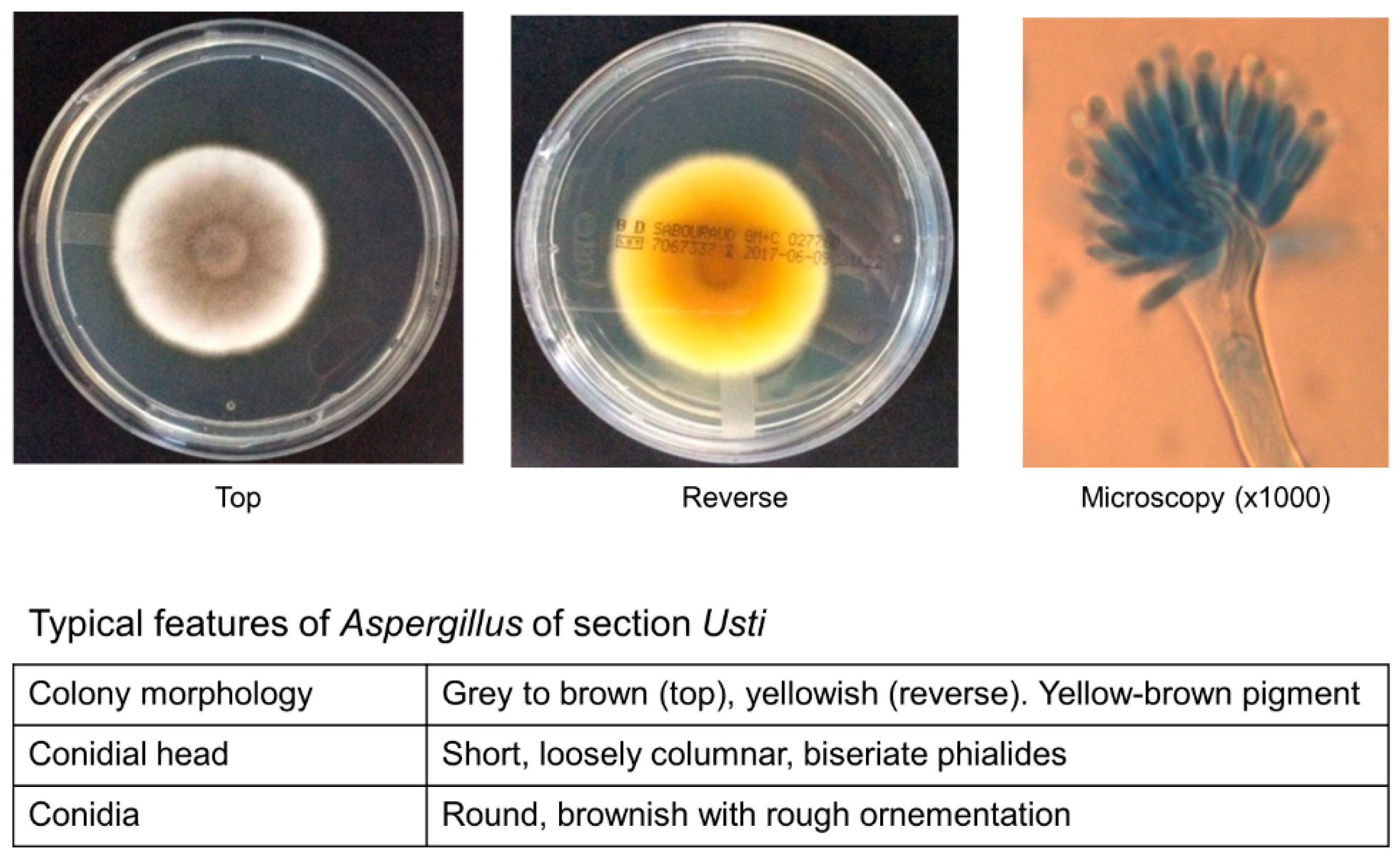The image features a triptych of square graphics, each showcasing a unique specimen presented in a clear circular dish against distinctive backgrounds. 

On the left, a dish set against a black backdrop contains a white circular specimen with a dark central spot, evoking the appearance of an eyeball, complete with a pupil and cornea-like structure, reminiscent of something observed under a microscope.

The middle graphic mirrors the first in layout but features a yellow specimen, also eye-like in appearance, contained within the same clear dish and black background, maintaining the theme of microscopic examination.

The rightmost square presents a blue, broccoli-like specimen in a clear dish, but switches to a pink background, offering a vibrant contrast to the previous images, while still adhering to the microscopic aesthetic.

Beneath these graphics, a rectangular chart provides detailed descriptions of each specimen in black text, offering further insight into the intriguing visuals above.